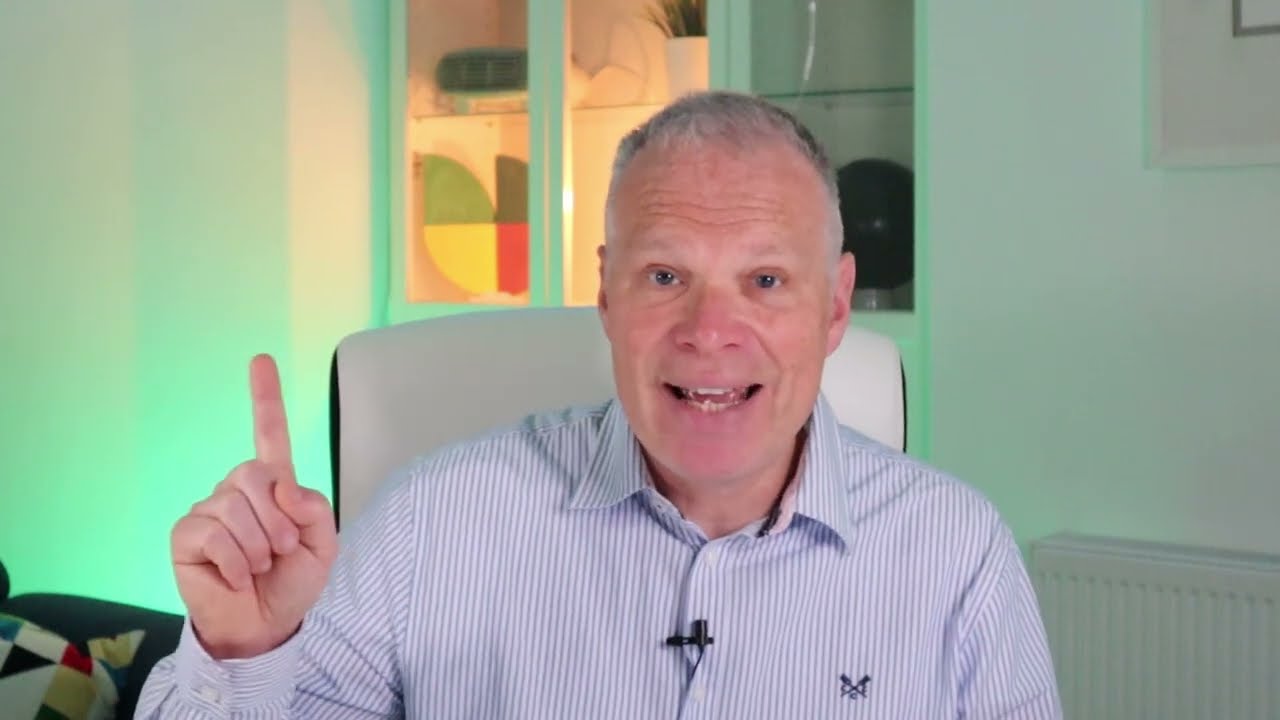In this photograph, an older man, likely in his 50s or 60s, is captured indoors, possibly in an office or a home setting filled with assorted objects. He sits centrally on a white chair, with a blue and white striped collared button-down shirt adorned by a small, clipped microphone. The man appears engaged, pointing his index finger upwards in a gesture that suggests he is making a point or delivering information. He wears an interested expression, accompanied by a smile that reveals his teeth. Behind him, the room is tinted with a greenish hue. A glass cabinet filled with various objects stands directly behind him, and a quilt-colored pillow, likely on a couch, is visible in the background. Additional objects, such as a wall heater in the bottom right corner and cushions or pillows in the bottom left, enhance the domestic atmosphere. The image seems to capture a moment in the middle of a video recording or presentation, as suggested by the man’s expressive demeanor and clipped microphone.